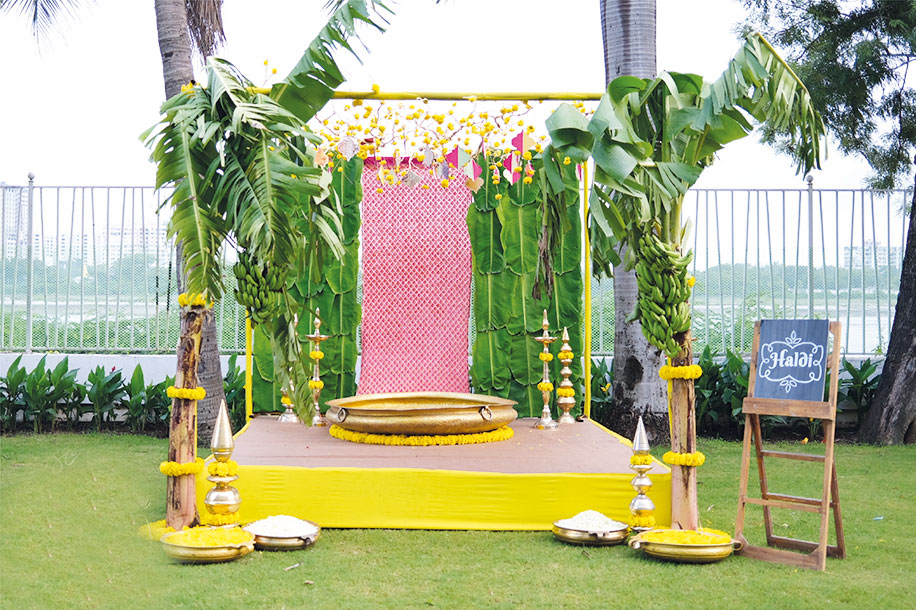The photograph captures an outdoor stage setup for a ceremonial event. The stage is a small platform adorned with yellow fabric on its sides and a hard brown surface on top. Dominating the back of the stage is a large brass pot with handles, positioned in front of a hanging red, see-through fabric that drapes from a bar. Flanking this red fabric are large green leaves, creating a natural curtain effect. Above this leafy curtain, a yellow bar festooned with multiple yellow flowers adds a festive touch. In the foreground, two large banana trees are planted at the front corners of the stage. Complementing the tropical vibe, more brass pots filled with salt and flower petals are positioned near the banana trees. The scene unfolds against an outdoor backdrop featuring a railing, a distant river, and buildings visible far off in the background, completing the picturesque setting. The vibrant colors in the scene include greens, yellows, browns, reds, whites, and several other hues, adding to the ceremonial ambiance.